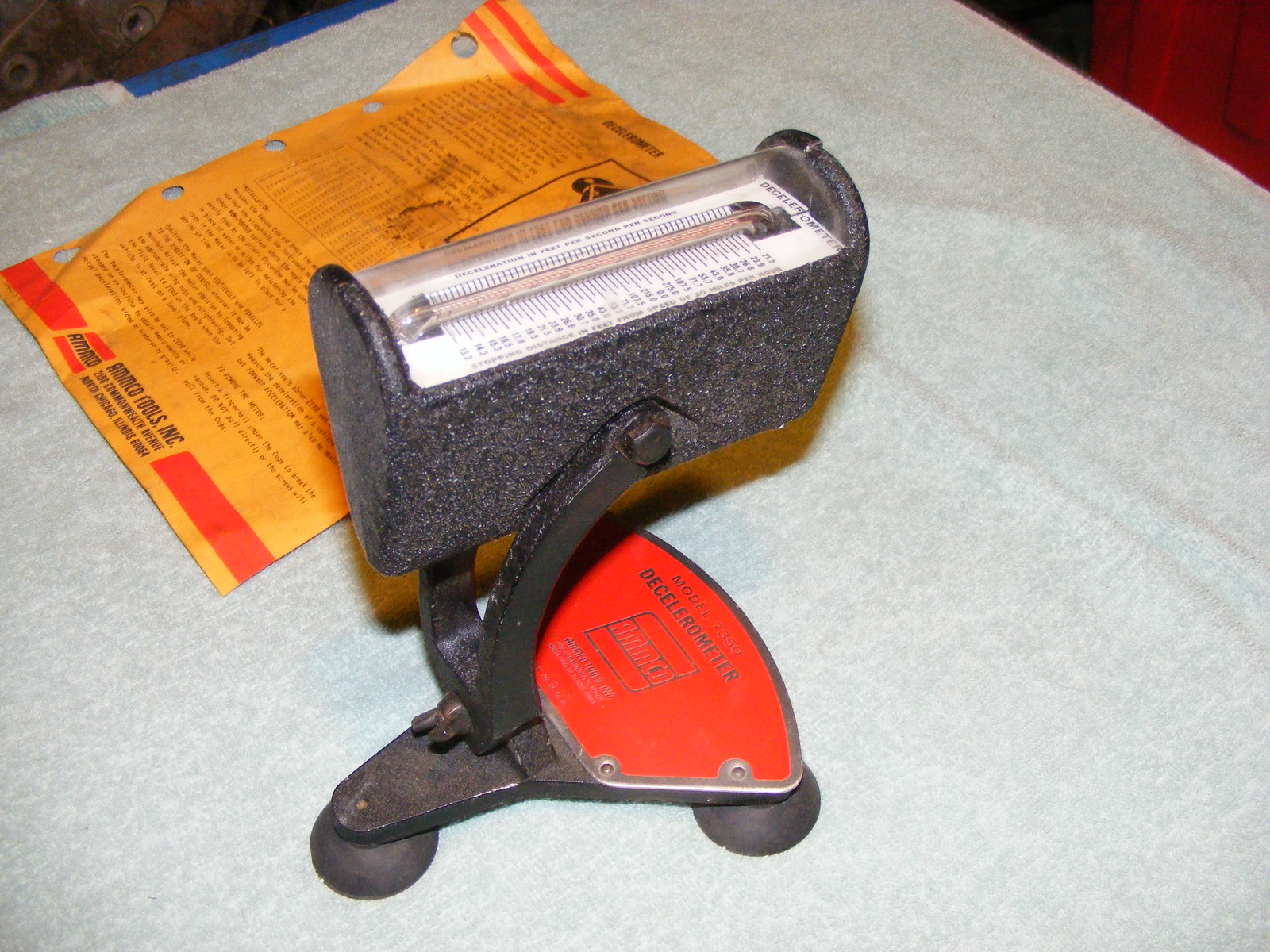The photograph features a detailed close-up of a gauge, depicted in a rectangular frame. The gauge itself is white and rectangular, fixed within a black surrounding frame. Prominently, it features a thin tube containing a red line, with numerous black numerical markings and notch lines on its white face. A protective round glass or plastic cover shields the gauge. It is mounted onto a distinctive curved Y-shaped bracket, which is affixed to a triangular base equipped with round feet at each corner for stability. A prominent metal plaque on the base reads in silver text: "Model 7850 AMCO Decellarometer." The base rests on a large gray and white towel. Adjacent to the gauge is an orange sheet of paper with several lines of black text, apparently providing instructions for the gauge's usage.